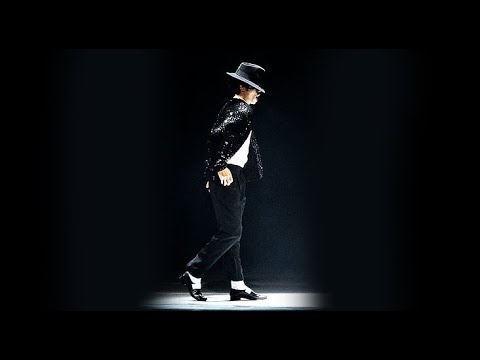In this striking photograph, Michael Jackson is captured mid-performance, embodying the essence of his iconic stage presence. Set against a completely black background, Jackson stands alone in the narrow beam of a spotlight, which illuminates his entire figure while everything else remains in shadow. He is dressed in his quintessential performance attire: a black fedora pulled low over his eyes, obscuring most of his face; a shiny, black jacket buttoned only at the top over a white shirt; black pants; white socks; and black heeled shoes adorned with white accents. His right hand, wearing his signature glove, is visible and positioned near his hip, while his left hand hangs by his side. Captured in mid-step, he appears to be either walking or performing his legendary moonwalk, with one foot planted firmly on the ground and the other sliding back. Jackson’s glasses add a final touch to this memorable image, which perfectly encapsulates his status as one of the greatest entertainers of all time.